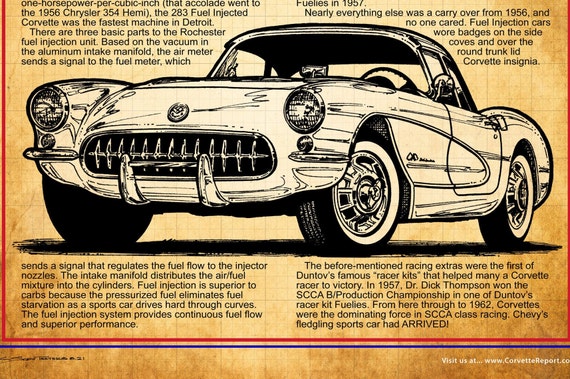The image is a vintage magazine advertisement featuring a detailed line drawing of an old-fashioned Chevrolet Corvette. Dominating the center of the page, the sporty two-seater car is illustrated in black and white with cream-colored details. It is set against a brownish-tan background, enhanced by a red border with a blue line underneath. The car is depicted with classic silver bumpers, headlights, and tires, resting on black pavement. Above the car's roof and below its tires, there is extensive text describing its specifications, design history, including mentions of the trunk lid, Corvette insignia, cylinders, and fuel injection. Notably, the text also highlights the model's historical significance, referencing the powerful 283 fuel-injected engine and its performance milestones in Detroit. At the bottom right corner of the poster, in white type, it directs viewers to visit www.corvettereport.com for more information.